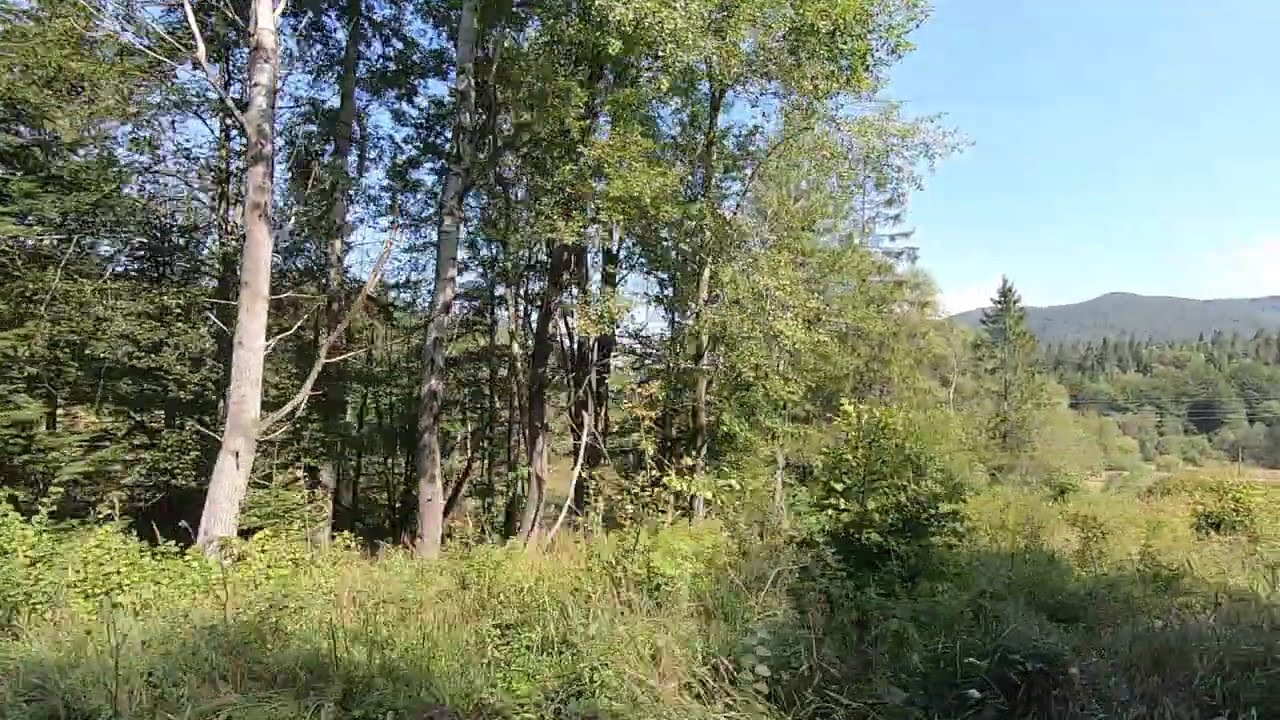This is a detailed and picturesque color photograph in landscape orientation, capturing a vast and serene forested area. The scene is dominated by a large stand of numerous green trees, mostly thin and tall, filling the left and center portions of the image. Overgrown grasses, bushes, and shrubs populate the foreground, adding to the lush, verdant feel of the scene. Toward the right side, there is a distant mountain range with a dark gray silhouette, creating a dramatic backdrop. Some power lines are visible in the background on the right, subtly cutting through the dense forest. The sky is a light blue with wispy, somewhat blurry clouds that suggest a partly cloudy but bright and sunny day, ideal for a walk though no visible trails are apparent. The forest is a mix of hardwoods and pine trees, with a row of smaller pines situated in front of the distant mountains. The image is a representation of photographic realism, capturing the natural beauty and expanse of this wooded landscape.